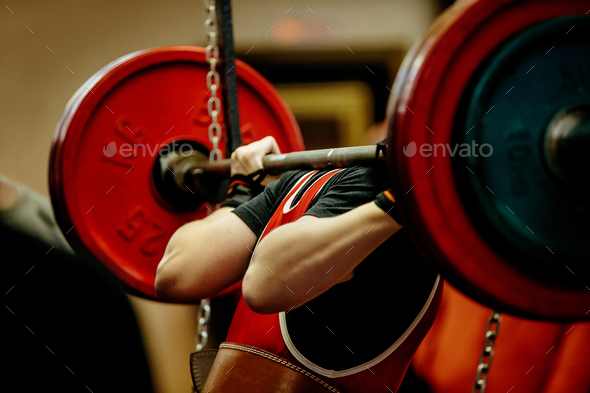The photograph captures a person, indistinguishable by gender, from the back, engaged in a weightlifting exercise. The individual is performing either squats or deadlifts, evident from the barbell positioned across their back and shoulders. They are adorned in a black short-sleeved T-shirt layered with a distinctive red tank top featuring white trim. A thick brown leather weightlifting belt secures their waist for added support. The person's hands grip the barbell, which is weighted with large red and black discs.

In the image, the person's head is obscured by the right-most weight, focusing attention on their upper body and the weights. The barbells are attached to a weight rack with silver link chains dangling on either side, ensuring the apparatus is stable. The background is a blurred mix of beige and black, hinting at a gym setting. Notable are the watermarks: 'Envato' appears at the center, overlaid with a checkered X pattern of dots across the entire image, adding a layered texture to the scene.